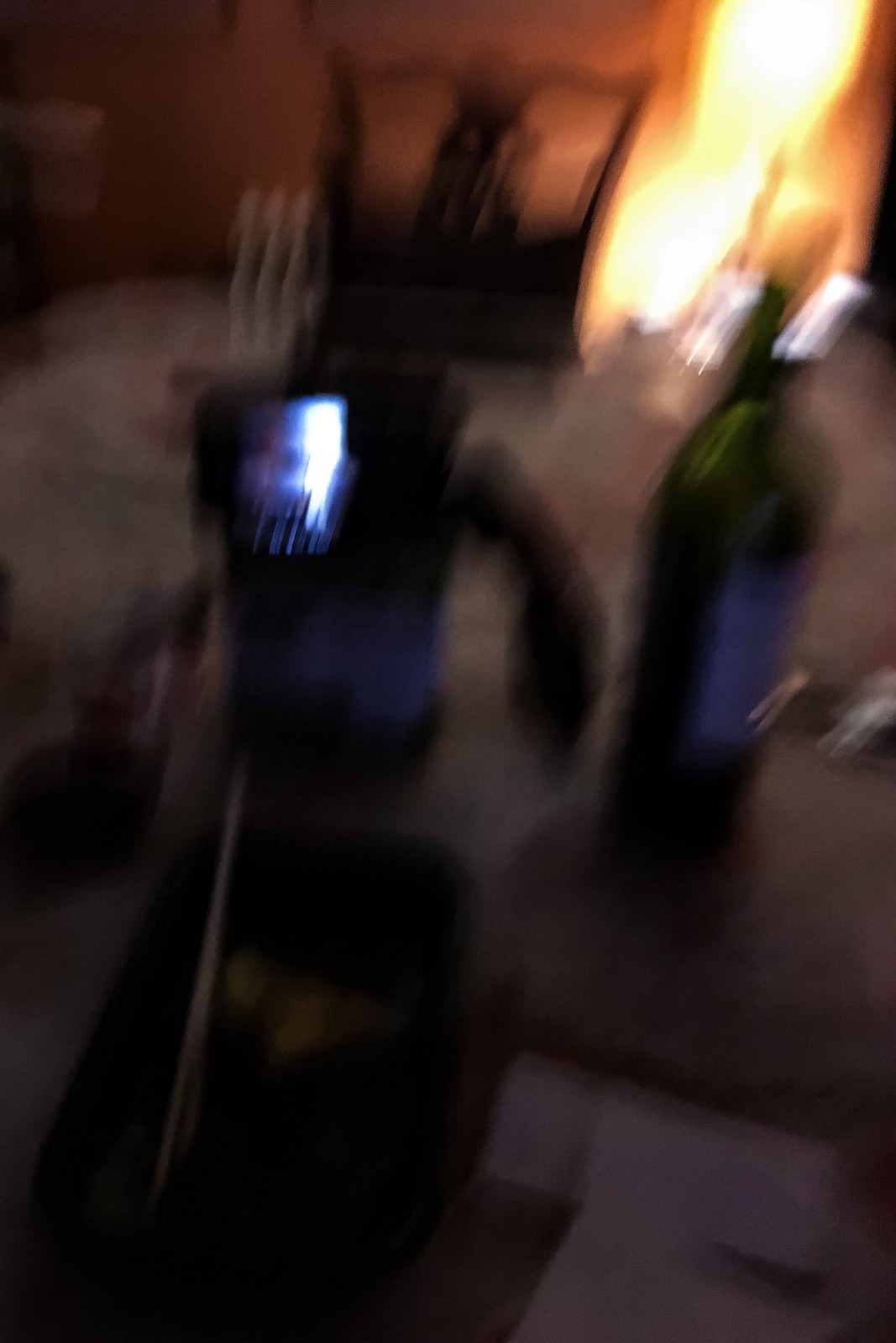The image is a blurry indoor shot, likely taken on a dining table. A prominent light source in the upper right-hand corner casts an orange glow over the scene, adding to the blur. To the left of the light source, there's a black object featuring two small vertical lines and a thick horizontal line at the bottom, possibly a chair or part of the furniture. In the foreground, a white surface holds a green wine bottle with a purple label placed beside a trash can. Directly in front of the camera are a stack of papers and plastic containers. The background reveals a piece of furniture that could be a cabinet or partially seen door or window, which allows light to flood into the room. There is also a dark tablecloth covering the table, making the scene dimmer except for the brightly lit spots. The overall ambiance is cluttered and dimly lit due to the reliance on natural light filtered through an unspecified source.